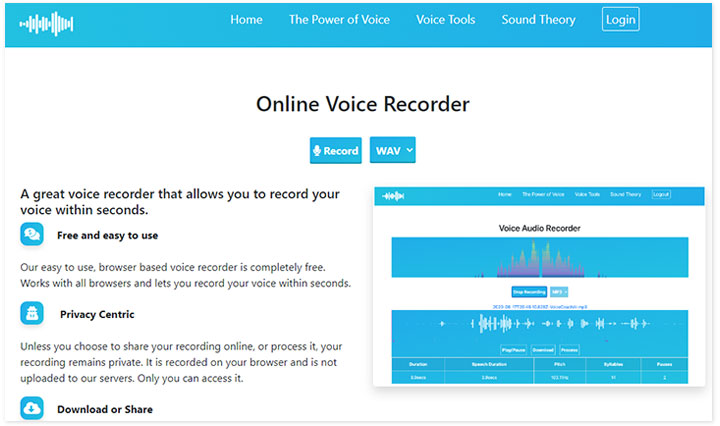This image depicts an online voice recorder webpage displayed on a computer screen. At the top, a light bluish teal banner showcases a voice pattern graphic on the left side. The banner also features navigation links labeled "Home," "The Power of Voice," "Voice Tools," and "Sound Theory." Towards the right end of the banner, there is a clickable "Log In" button enclosed in a white rectangle.

Centered on the page, in bold black print, the headline reads "Online Voice Recorder." Directly below, a blue rectangle containing the word "Record" invites users to start recording. Adjacent to the record button is a dropdown menu labeled "WAV," allowing users to select their desired audio format.

On the left side of the page, a section highlights the tool's primary features with the text: "A great voice recorder that allows you to record your voice within seconds." An accompanying speech bubble icon emphasizes that the tool is "free and easy to use." Further down, another blue bubble with the label "Privacy Centric" is followed by a paragraph detailing the tool's privacy features.

Towards the bottom of the screen, a download cloud icon accompanied by the text "Download or Share" indicates options for handling recorded audio files. On the right side of the image, part of the voice recorder interface is visible.